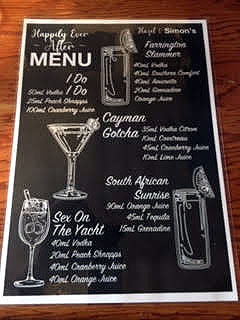This image features a wedding menu elegantly placed on a rustic wooden table. The menu's design is sophisticated, with a sleek black background, a crisp white border, and stylish white text. Emblazoned at the top, the words "Happily Ever After" set a romantic tone, followed by the heading "I Do," which introduces a curated list of specialty cocktails.

Underneath this heading, several enticing drinks are listed: 
- "Cayman Gapja," 
- "South African Sunrise," 
- "Sex on the Yacht."

Each drink is accompanied by illustrations of different glasses that reflect their unique presentations. A martini glass stands poised and elegant, a wine glass is depicted with ice and a straw, and a cocktail glass features playful lime wedges in its corners. Notably absent are any prices, hinting at a celebratory, no-expense-spared evening. The image captures only the menu itself, focusing on the details of the drink offerings with no people or additional elements visible in the frame.